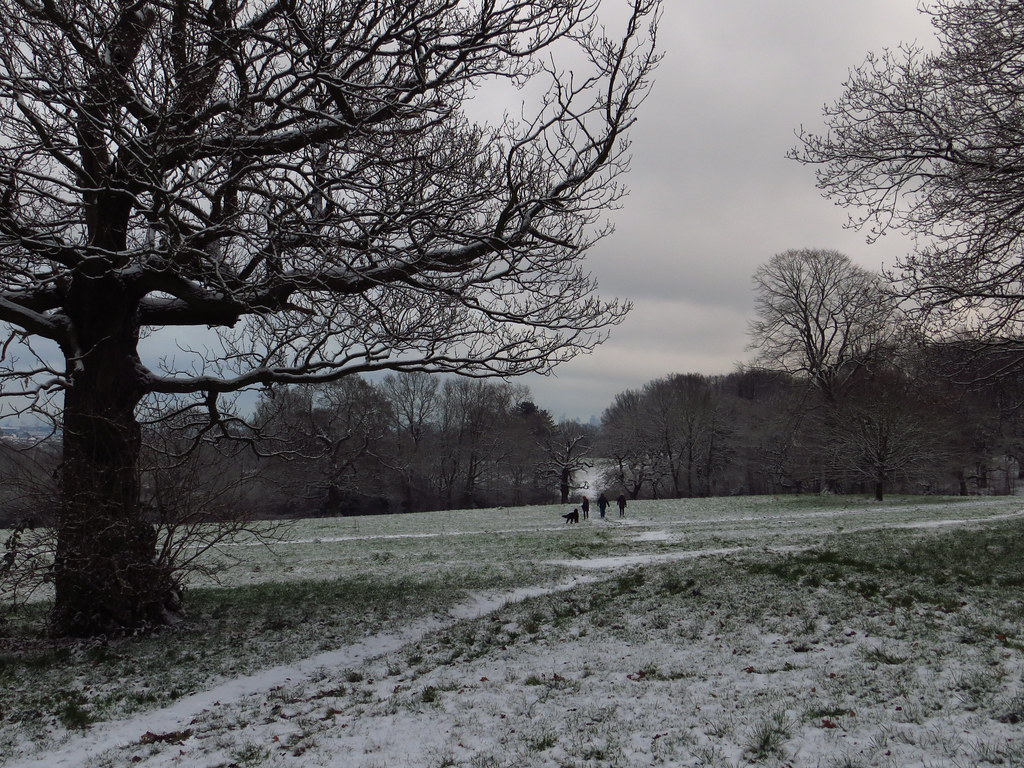The image captures a wintry outdoor scene in a park or farm, likely taken during early winter or late fall. The landscape features a mix of frosty and lightly snow-covered ground, with patches of exposed brown and green grass. The sky is overcast with thick, gray clouds, hinting at an impending dusk. 

Dominating the left side of the image is a large, leafless tree, its bare branches reaching skyward. To the right and toward the background, a line of trees stands at the edge of what appears to be a river, with more trees visible across the water. These distant trees are also stripped of their leaves, adding to the stark, chilly atmosphere. 

Near the center-right of the scene, three people are walking with a large black dog, their figures appearing almost as silhouettes against the wintry backdrop. The ground around them is frozen, and a light layer of snow clings to the branches above. The picturesque yet cold outdoor setting evokes the serene stillness of a late afternoon in winter, as the sun begins its descent.